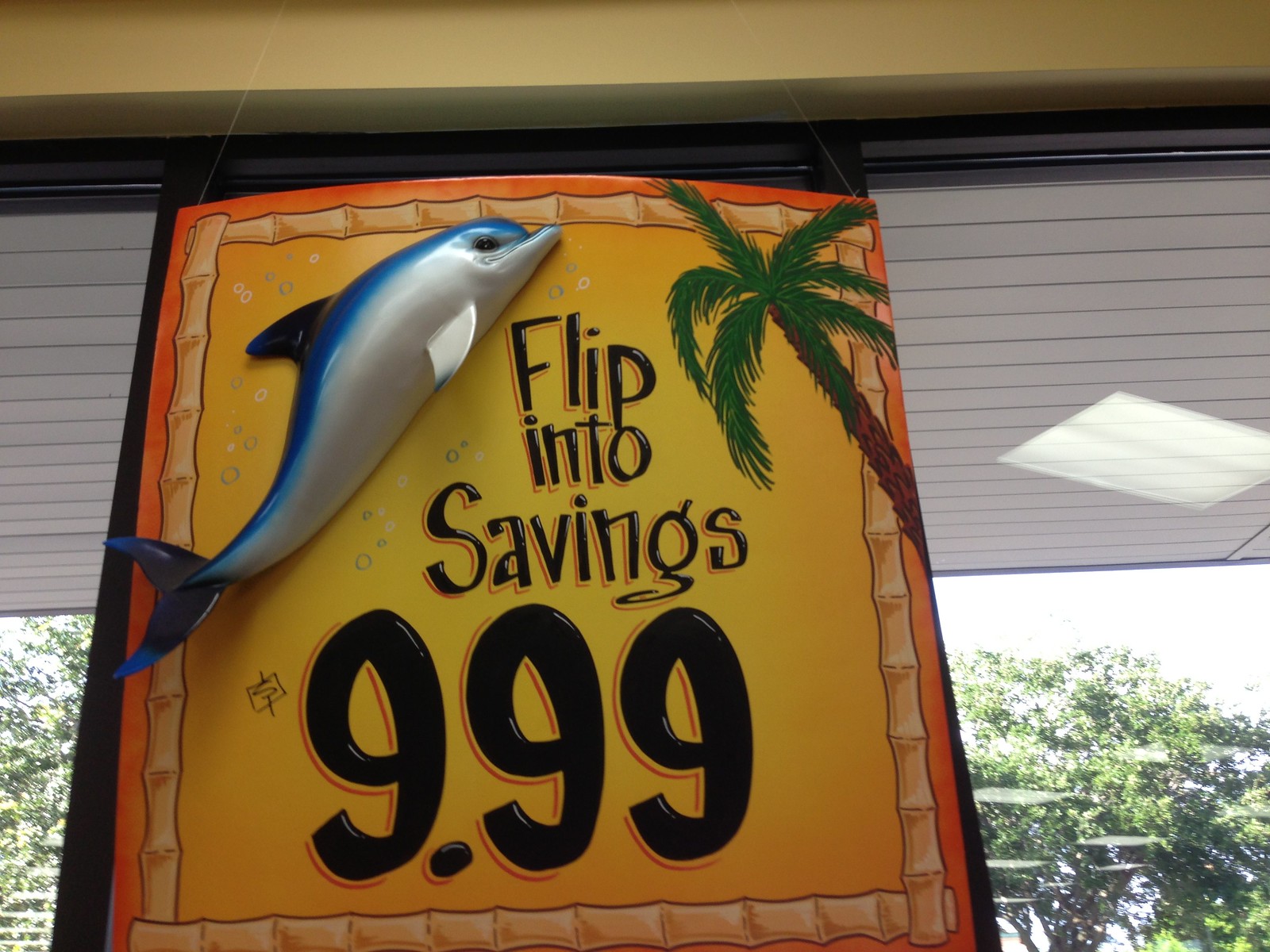The image captures a detailed poster advertisement mounted inside a store window, framed by black metal window panes that offer a glimpse of the outdoors and a beige wall above. The poster itself commands attention with its vibrant orange and lighter orange hues, outlined by what appears to be bamboo shoots on all corners, creating a cohesive and naturalistic border. Dominating the top portion of the poster is a three-dimensional plastic model fish—blue on top with a white underbelly, fins on the sides, and a blue tail—that could be mistaken for a dolphin or shark. The bold black text in the middle of the poster reads "Flip into Savings," emphasizing the central message against the colorful backdrop. Beneath this, the eye is drawn to the prominently displayed price of $9.99. In the bottom right corner, a palm tree leans diagonally toward the center, adding an island vibe to the display. The poster is situated in a large window, through which multiple trees outside are visible, along with the reflection of an overhead light on the partially raised blinds, enhancing the depth and realism of the scene.